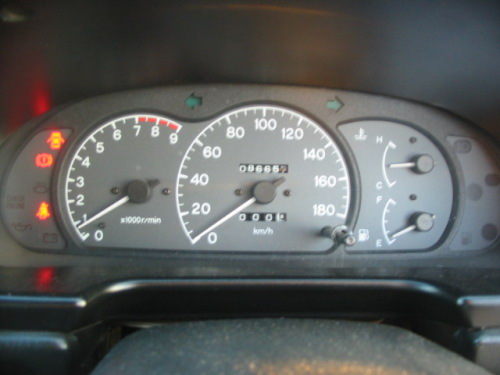A photograph taken from inside a vehicle captures an intricate view of the gauge cluster from the driver's perspective. On the left side of the cluster, the RPM gauge is prominently displayed, ranging from 0 to 9, with the 7 to 9 range marked in red, indicating the danger zone. Below, the gauge is labeled "x1000 R/min." The central gauge displays the speedometer, calibrated in kilometers per hour from 0 to 180, in increments of 20. Notably, the odometer in the middle shows a reading of 86,657 kilometers. On the right side, two smaller gauges are present; the top one indicates the engine coolant temperature, labeled from 'H' for high to 'C' for cool, while the bottom gauge shows the fuel level, marked from 'F' for full to 'E' for empty. Additionally, green signal lights are visible at the top of the cluster. The entire image is framed in a rectangular shape, providing a clear and detailed view of the vehicle's instrumental panel.